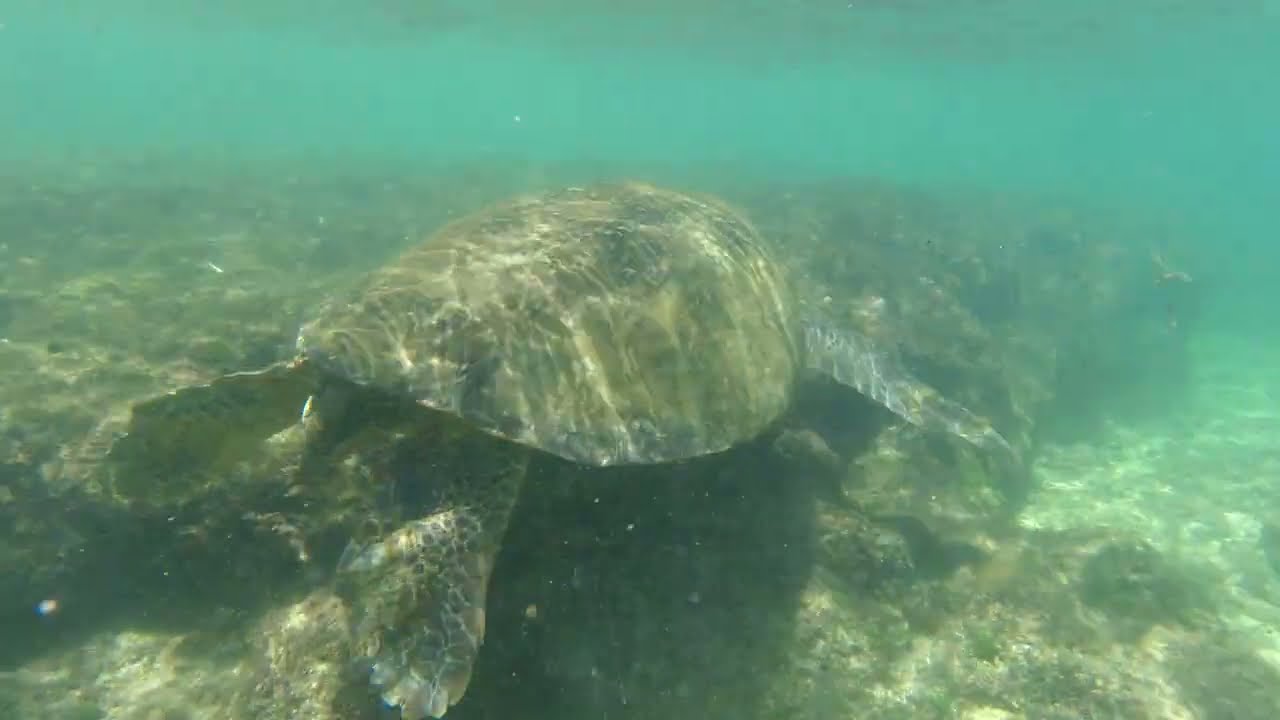This underwater photograph captures the back of a large sea turtle swimming through murky aqua blue water. The image is slightly cloudy, with a predominantly greenish tint. The turtle, swimming to the right and slightly upward, appears to be moving away from the camera over a rocky ledge or reef area that spans across the image. The turtle’s dark brown shell with a distinctive black spot on top is visible, as well as its right front fin and two back feet trailing behind. The head of the turtle is obscured from view. The ocean floor in the foreground features various rocks, and the rocky ledge creates a step-down effect to a lower level, blending almost seamlessly with the surrounding water. The upper part of the photograph fades into the murky, aqua blue water, adding to the sense of depth and the turtle's journey through its underwater habitat.